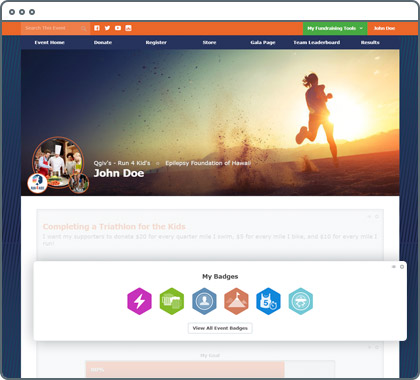A screenshot of a small tablet displays a vibrant interface. An orange bar spans the top of the screen, featuring search options for Facebook, Twitter, and two other unidentifiable social media platforms due to their small icons. Below this, a prominent green section displays text in French, though the specifics are unclear.

Within this green block, six clickable options are available. Below the options, an image showcases a runner in a desert-like environment, with sand spraying from their feet as they speed along. To the right, the sun is either setting or rising, casting dramatic light on the scene.

On the left, there's an icon depicting a chef in a tall hat, assisted by another person, preparing food. This section is labeled "John Doe" and highlights achievements in a triathlon event, indicating participation and badge awards. The combination of a runner and a chef seems to correlate with different aspects of the user's activities or interests.